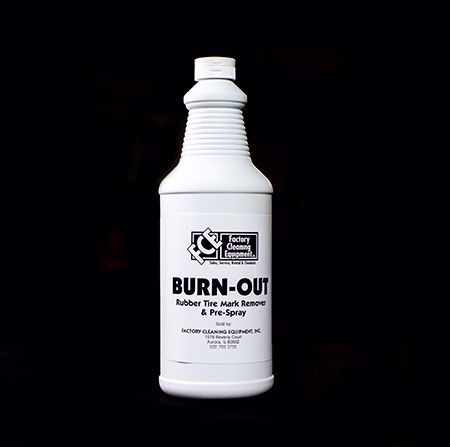The photograph features a white, cylindrical plastic bottle with a small white cap and a ribbed neck for improved grip. The bottle stands against a black background and prominently displays text in bold black letters. The main label on the bottle reads "BURNOUT," referring to the product name, with an additional description underneath: "RUBBER TIRE MARK REMOVER AND PRESPRAY." At the top of the bottle is a rectangular label with the logo "FCE" in diagonal lettering, representing Factory Cleaning Equipment. To the right of the logo, the text reads "FACTORY CLEANING EQUIPMENT." The bottom part of the bottle contains smaller black text, providing an address and additional information, which is difficult to read. The overall design is clean and professional, emphasizing the bottle's purpose as a specialized cleaning solution.